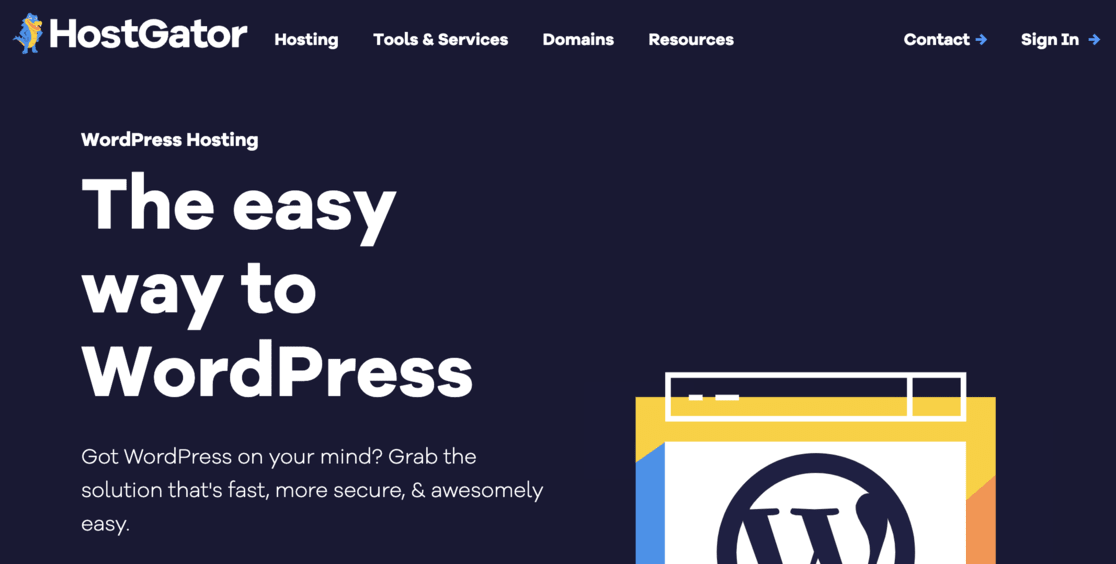In this promotional image set against a sleek black background, bold white text in the upper left corner reads "HostGator." Adjacent to this text is the HostGator logo, featuring a cheerful alligator in blue and yellow standing upright with its front legs placed confidently on its hips. To the right of the logo, a navigation bar lists key options: "Hosting," "Tools and Services," "Domains," "Resources," "Contact," and "Sign In."

Below the navigation, large text proclaims "WordPress Hosting," followed by "The Easy Way to WordPress." A tagline urges, "Got WordPress on your mind? Grab the solution that's fast, more secure, and awesomely easy."

On the right-hand side of the image, there is a three-dimensional graphic of a box. The front face of the box is white, prominently displaying the top of a "W" enclosed in a circle, symbolizing WordPress. The promotional text is reiterated next to the box, underscoring the ease and security of HostGator's WordPress hosting services.